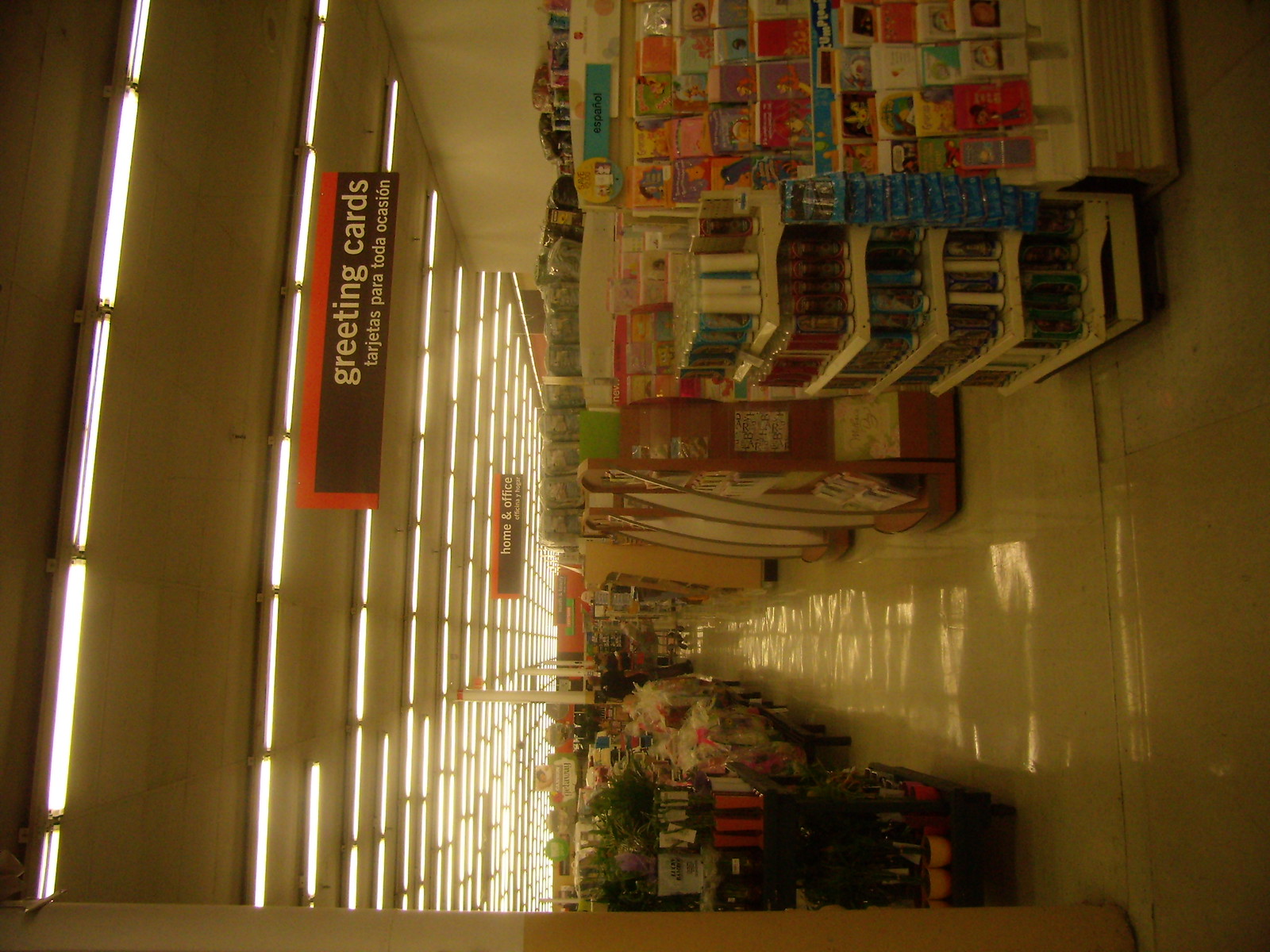The image captures a slightly tilted view of a store interior, giving it a unique perspective. The lighting appears unusual, casting a brownish hue over the scene, possibly due to a filter. Despite numerous ceiling lights, the ambiance still feels dim. On the left side of the image, there is a sign that reads "Greeting Cards" in white text, with a Spanish translation beneath it, all set against a black or dark brown background with an orange border. Upon zooming in, one can spot tall, white candles adorned with intricate paintings and drawings. Additionally, there's a distinct section marked "Español," featuring an array of greeting cards, including one with a Winnie the Pooh design, likely intended for various special occasions.